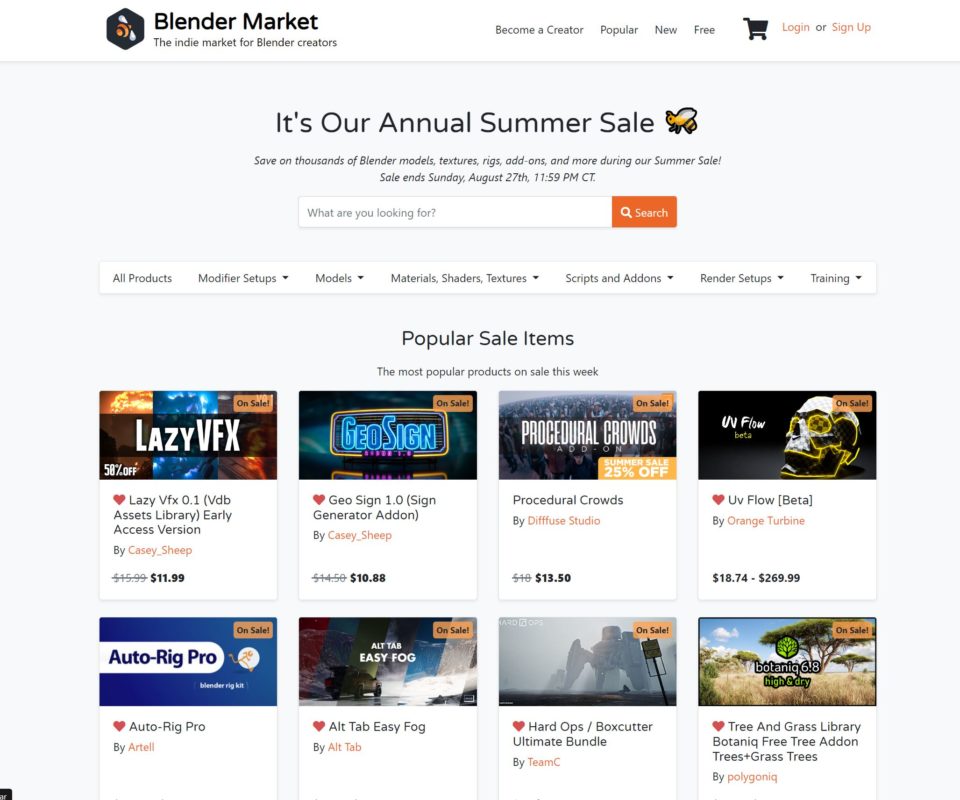This image depicts a promotional banner from Blender Market, an online marketplace dedicated to Blender creators. Blender, a free and open-source 3D graphics software, is popular among filmmakers, game developers, and digital artists for creating 3D animations, models, and more.

The banner features a light gray background and a prominent search bar. The focal point of the banner is an announcement about the annual summer sale, stating, "Save on thousands of Blender models, textures, rigs, add-ons, and more. Sale ends August 27th." 

Several featured items are highlighted, including:
- LazyVFX, priced at $12
- GeoSign, priced at $11
- Procedural Crowds, priced at $13.50

Additionally, a product titled "Tree and Grass Library" is visible, showcasing resources that help creators streamline their work by not having to start from scratch. The market positions itself as an indie platform, appealing particularly to independent developers and artists who often work with tighter budgets.